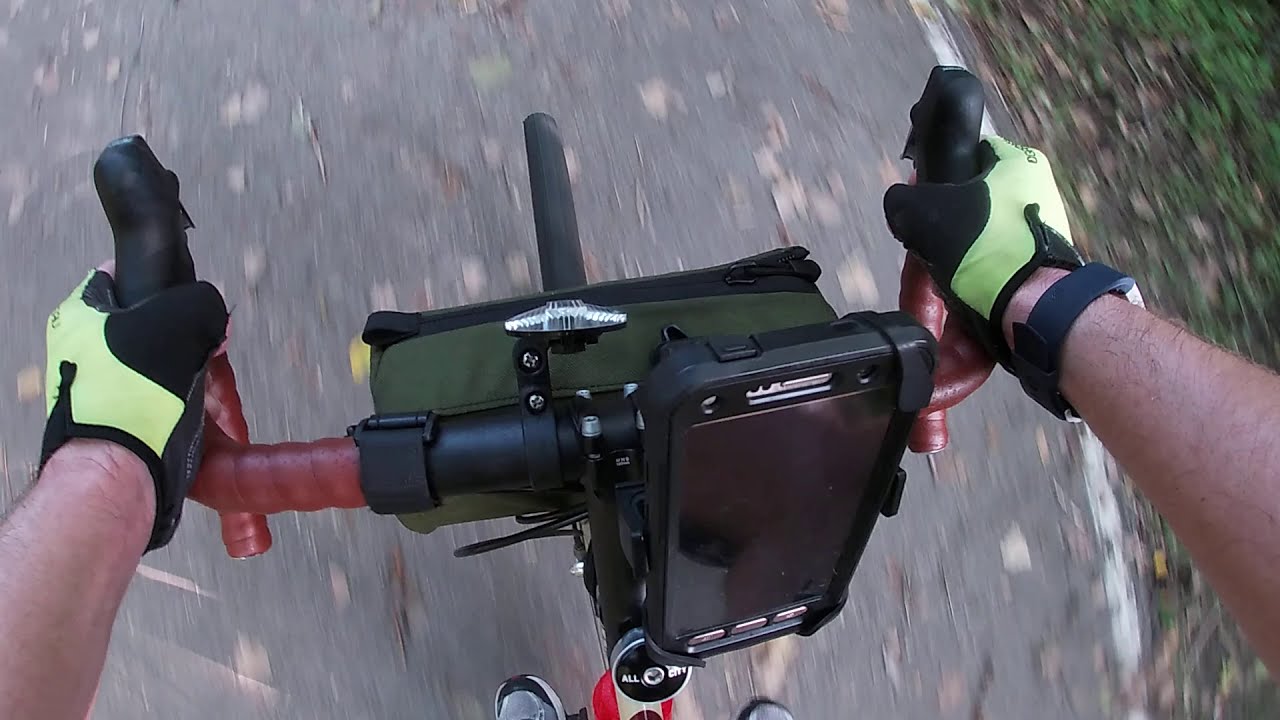The image, captured from the perspective of a cyclist's helmet cam, presents a vibrant, motion-filled scene of a ride on a red bike. The cyclist, possibly male, wears black and lime green gloves and sports a black smartwatch on their right arm, which is notably hairy. Their arms extend from the lower part of the image towards the center, holding onto red handlebars. A smartphone is mounted between the handlebars in a holder, overshadowed by a green zippered pouch in front of the handlebars. The view also includes the top of the front tire and the blurred pavement underneath, indicating significant speed. The paved path is lined with some dirt and small plants on the right side, while the rest of the ground, peppered with some leaves, is bathed in natural daylight. At the bottom of the photo, the tips of the cyclist's shoes are just visible, further grounding the perspective in dynamic motion.